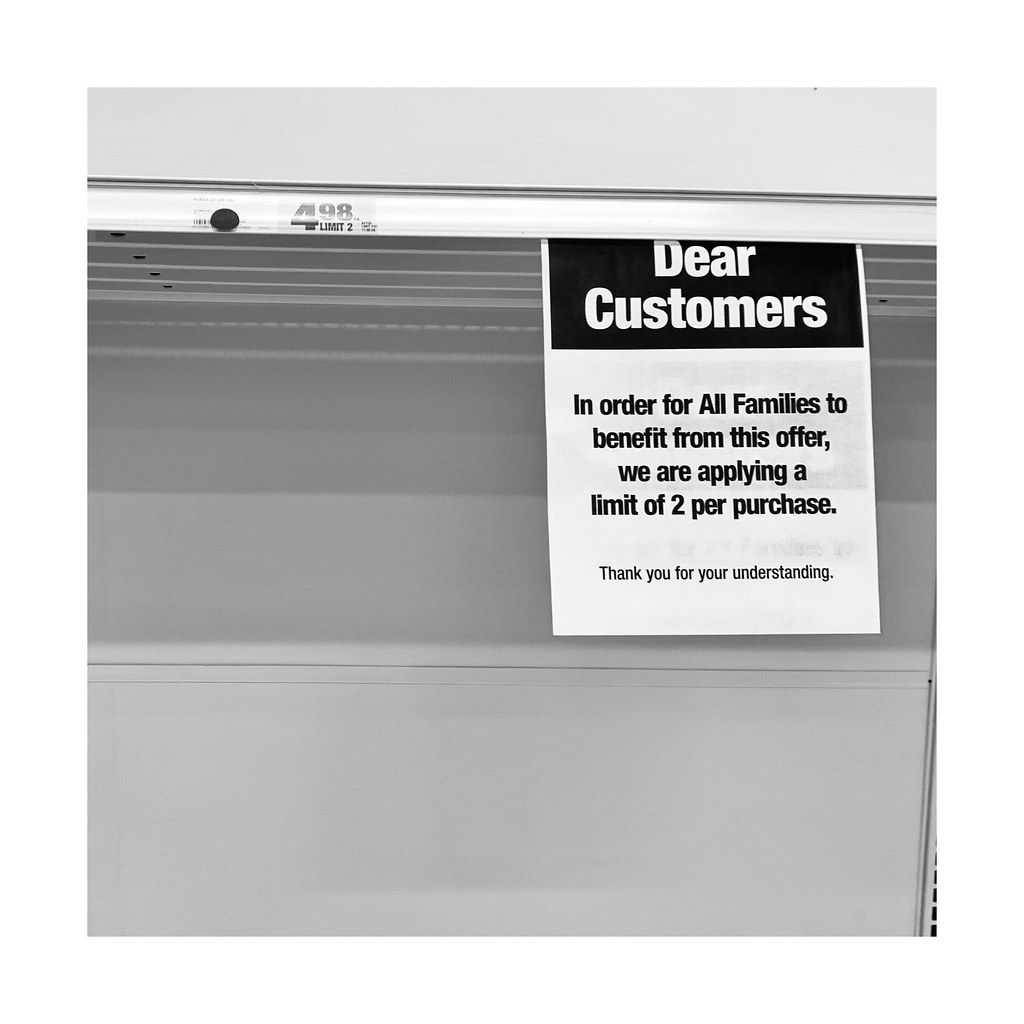This detailed grayscale photograph showcases an empty shelf in a store, metallic light-gray due to shadowing and varying shades of gray in the background. The shelf prominently features a price tag displaying "$4.98, limit 2." Positioned near the tag is a standard 8x11 inch sheet of printer paper with a printed notice in big, bold letters: "Dear Customers." Beneath this heading, the sign states, "In order for all families to benefit from this offer, we are applying a limit of two per purchase. Thank you for your understanding." Both the price tag and the notice emphasize the purchase limit. Despite the intended offer, the shelf is entirely bare, void of any products for purchase.